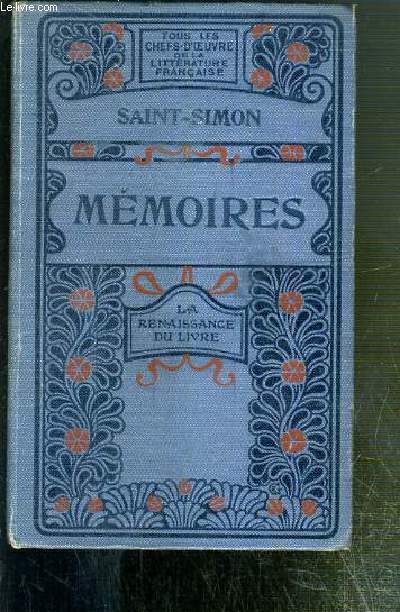The photograph showcases an intriguing cover of a French book or diary titled "Saint-Simon Mémoires." The central part of the cover prominently displays the word "Mémoires" alongside the words "La Renaissance du Livre," indicative of a classic or historical publication. In the top left corner, the website "LeLivre.com" is written in white font. The overall background color of the cover appears to be a blend of dark blue, light blue, and black, adorned with an elegant orange floral pattern. This book cover dominates the vertical rectangular image, occupying most of the space and is slightly positioned to the left. The setting seems to be indoors, with the book resting on a surface that appears to be a forest green table or background. The entire scene evokes a vintage yet sophisticated aesthetic.